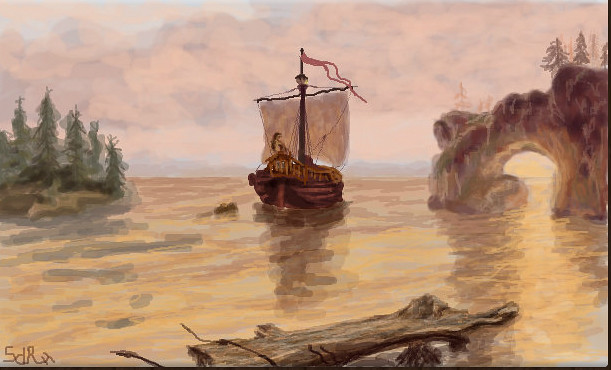A stunning piece of artwork captures a ship sailing gracefully in the ocean, positioned centrally within the composition. The ship, constructed from rich brown timber, features a prominent brown mast adorned with a slender red flag fluttering at its peak. A large, white rectangular sail billows in the wind, propelling the vessel forward. The painting, rendered in either watercolors or oil paints, is awash with the warm and vibrant hues of a sunset, blending yellows, oranges, pinks, and soft blues to create a serene, dreamlike atmosphere.

In the foreground, a solitary log rests on the right side of the scene, adding a touch of realism and depth. To the right, the coastline is marked by a rugged rocky arch, while to the left, a cluster of verdant green fir trees stands tall, their lush branches contrasting against the warm tones of the sky. The combination of these natural elements with the central ship creates a balanced and harmonious composition, inviting viewers to lose themselves in the tranquil beauty of this maritime journey.